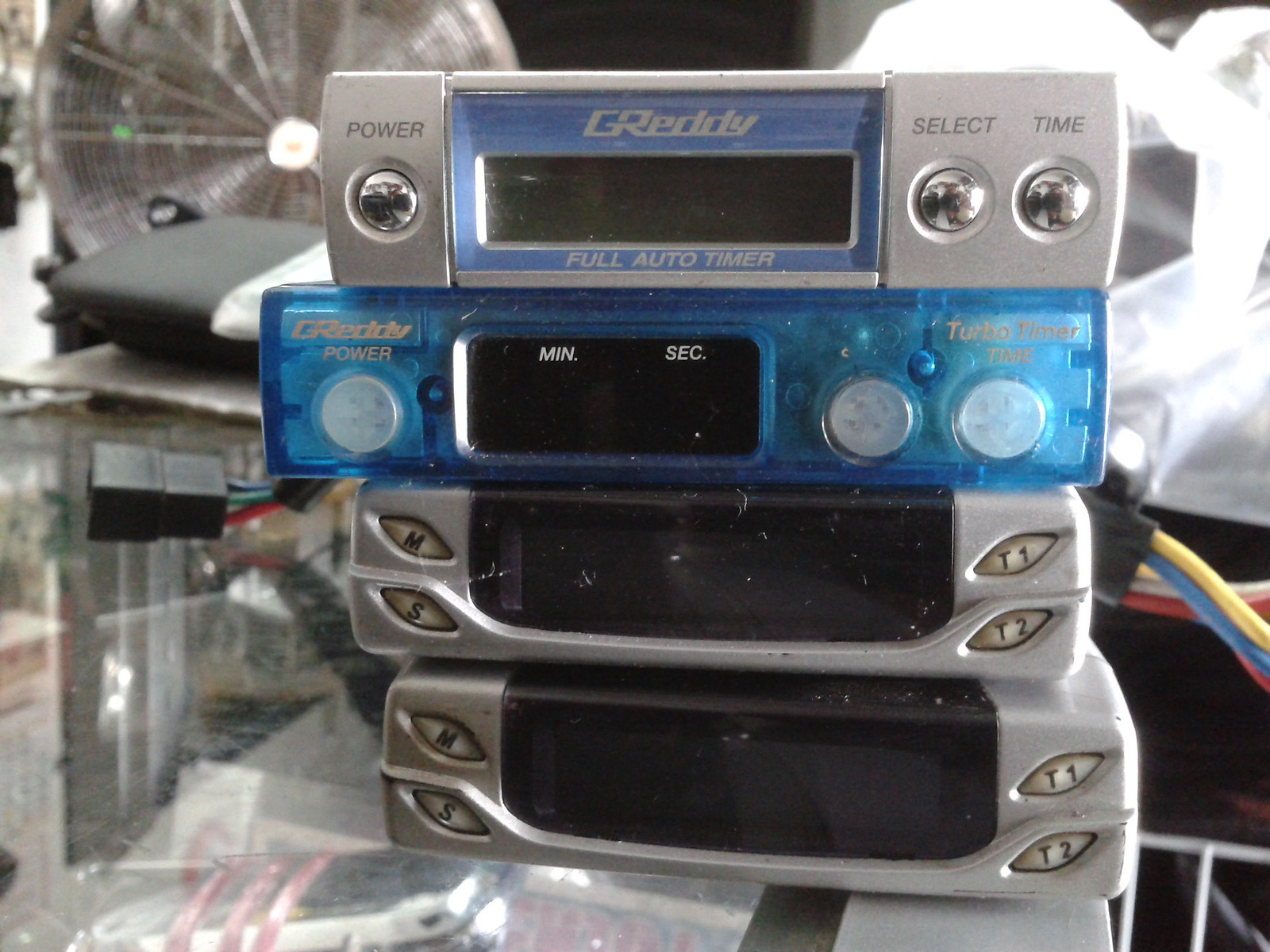The photograph showcases a stack of four vintage electronic timers, seemingly from the 1980s or 1990s, arranged on a glass surface. The two bottom timers are identical with gray casings, featuring prominent black rectangle displays and diamond-shaped labels denoting "M" for minutes, "S" for seconds, and buttons labeled "T1" and "T2" on the right side. Above these, there's a blue-cased timer labeled "Greddy Turbo Timer," which displays minutes and seconds on its central screen. On the left side, it has the markings "Greddy" and "Power." Topping the stack is a silver timer with a blue rectangle display inscribed with "Greddy Full Auto Timer." This top timer has a circular power button on the left, along with select and time buttons, featuring a more metallic finish than the others. The background reveals a blurry fan and some cables, adding to the vintage technological ambiance of the scene.